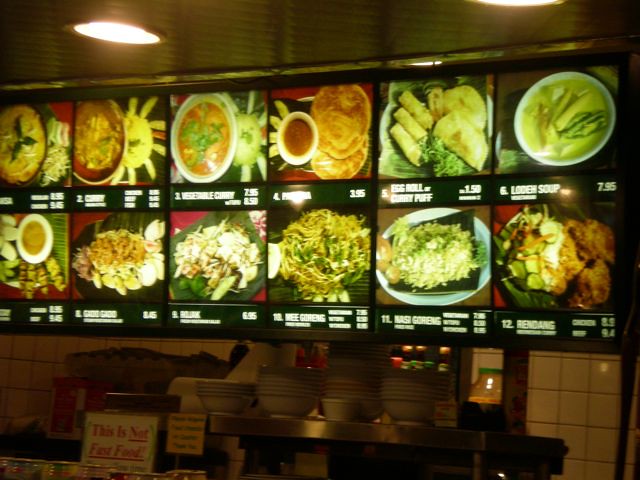Photograph Description:

In this vibrant photograph, we are presented with the bustling front counter of an Asian restaurant. Above the opening to the kitchen area, a brightly illuminated menu showcases an array of delectable dishes. The menu board displays a total of 12 items, although only a few are clearly legible. Among the highlighted selections are "Egg Roll" and "Loaded Egg Roll" priced at $1.50 each, "Loaded Soup" for $7.95, "Rendang Chicken" at $8.98, and "Rendang Beef" for $9.00. The remaining items are partially obscured and not entirely readable.

A prominent sign beneath the menu states, "This is not fast food," emphasizing the restaurant's dedication to quality and authenticity. Below the sign, a stainless steel shelf holds an array of bowls, hinting at the preparation of fresh dishes. The background is adorned with traditional ceramic tiles, adding to the establishment's authentic and cozy atmosphere. 

This detailed scene captures the essence of an inviting Asian restaurant, enticing patrons with its illuminated display and promise of delicious, carefullycrafted meals.